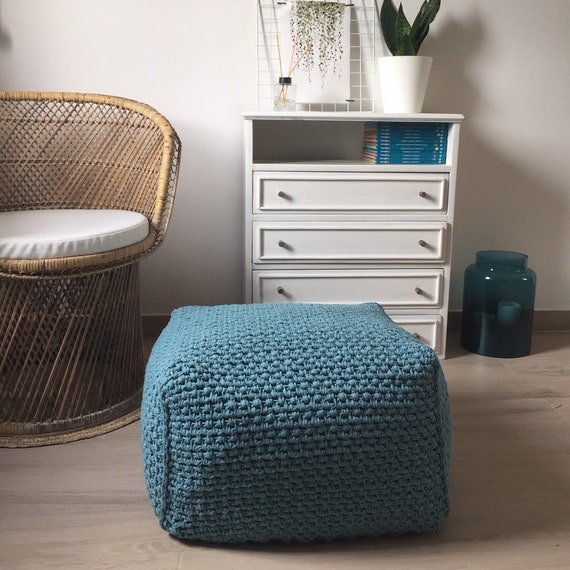This color photograph depicts a cozy bedroom with a light and airy ambiance. Dominating the room is a white chest of drawers featuring four drawers, each adorned with black knobs. Above the top drawer is an open shelf neatly housing a stack of slender, green books, which appear to be around twenty in number. Atop the chest, there is a decorative white pot holding a thriving green plant, alongside what seems to be a small diffuser with three reeds protruding from it. Adjacent to these is a blue glass container, likely a candle holder, adding a touch of elegance to the setup. Reflecting the scene behind the chest is a mirror, further enhancing the room's spacious feel.

In the foreground rests a blue ottoman, its knitted or fabric cover contributing a soft, cozy texture to the space. The ottoman provides a pop of color against the light tan hardwood floor, which is visible and showcases its beautiful grain. To the left of the chest of drawers stands a wicker chair with a unique round, legless base and a white round cushion, perfect for relaxing. The chair's handmade, tropical aesthetic adds warmth and character to the room. These elements together, against the backdrop of white walls and subtle crown molding, create a harmonious blend of blues, whites, and natural tones, making the room feel welcoming and well-balanced.